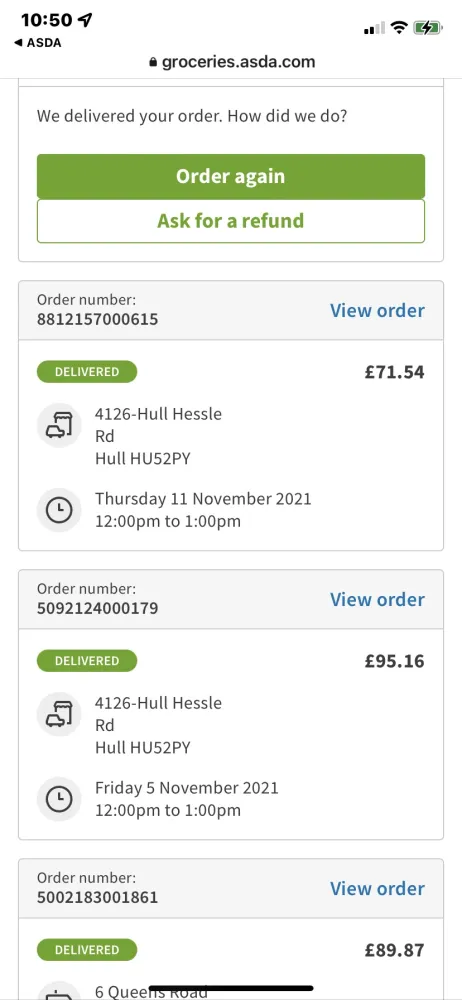A detailed description of the image showing a mobile version of a grocery website order summary page:

The image displays a screenshot of the mobile version of a website, groceries.azda.com, specifically on its order summary page. At the top of the page is a prominent box featuring a customer feedback prompt: "We delivered your order, how did we do?" Within this box, two distinct buttons are placed beneath the prompt. The first button is green with white text that reads "Order Again," and directly below it, there is a white button with green text that says "Ask for a Refund."

Underneath this feedback section, the screen shows a series of detailed order cards, each representing a previously delivered order, sorted by their delivery dates. The first order card, located immediately beneath the feedback box, is designated with the order number 8812157000615. The card features a "View Order" button on the top right corner, alongside comprehensive information including the total pricing, the status labeled as "Delivered," the delivery address, and the delivery time.

Following the first card, the second order card is labeled with the order number 5092124000179, maintaining a similar layout and set of details. The third card presents the order number 5002183001861. Each card indicates pricing in pounds, signifying the UK origin of the website. Overall, the image provides a clear view of the order summary page, emphasizing the user-friendly design and thorough information provided for each order.